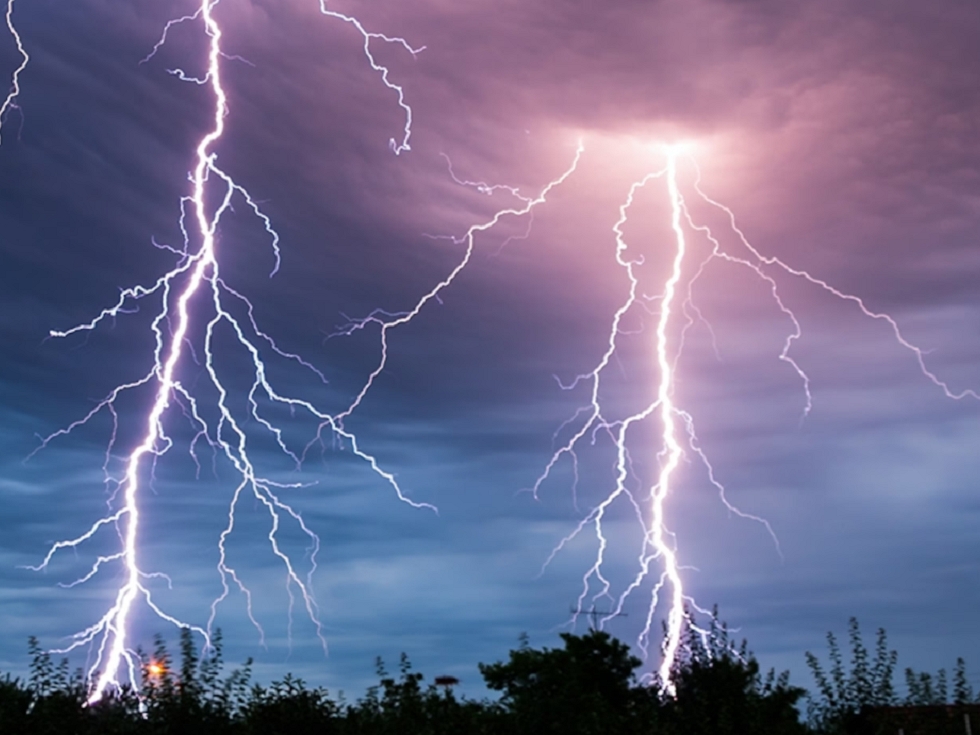This stunning photograph captures a rare and dramatic display of nature's power, featuring multiple lightning strikes against a purplish-blue, smoky sky. Two main lightning bolts, positioned side by side, dominate the image, with their branching arms slicing through the clouds and reaching down towards the silhouetted trees and plants below. The top half of the sky is painted in shades of lavender purple, which seamlessly fade into dark and light blues, creating a striking backdrop. The lightning appears to emerge from the clouds, with intricate veins and lines clearly visible as they descend. The bottom of the photo shows the tops of darkened trees, and in the distance, an electrical pole and a faint street lamp can be seen, adding to the moody, atmospheric quality of the scene. The angle of the shot, taken looking upwards, enhances the grandeur and scale of the lightning, making it one of the most beautiful and unique images of its kind.